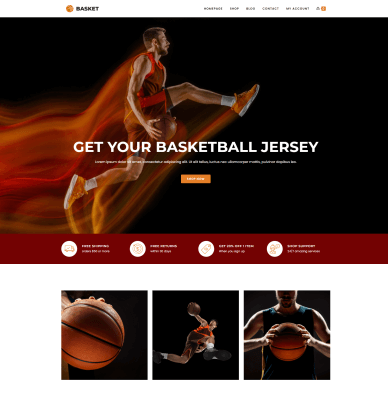In this image, we see a detailed screenshot featuring an AI-generated depiction of a basketball player. The player is captured in an action pose with his left leg raised and right leg grounded, facing east. His right hand firmly grips a basketball while he dons an orange uniform, enhanced with dramatic flames emanating from his back, adding a dynamic energy to his form. Overlaying the top of the image, there is a bold white text that reads, "Get your basketball jersey." Just below this text, an orange action button invites user interaction. Below the button are three vivid photographs, each illustrating different aspects of basketball. The lower-left photo provides a close-up of a basketball; the center image shows the same player soaring through the air with his legs kicked up, and his right arm extended above him holding the basketball; the final photo on the right offers a waist-up close-up of the athlete, both hands securely holding the ball. This composite of visuals and text effectively evokes the excitement and dynamic nature of basketball.